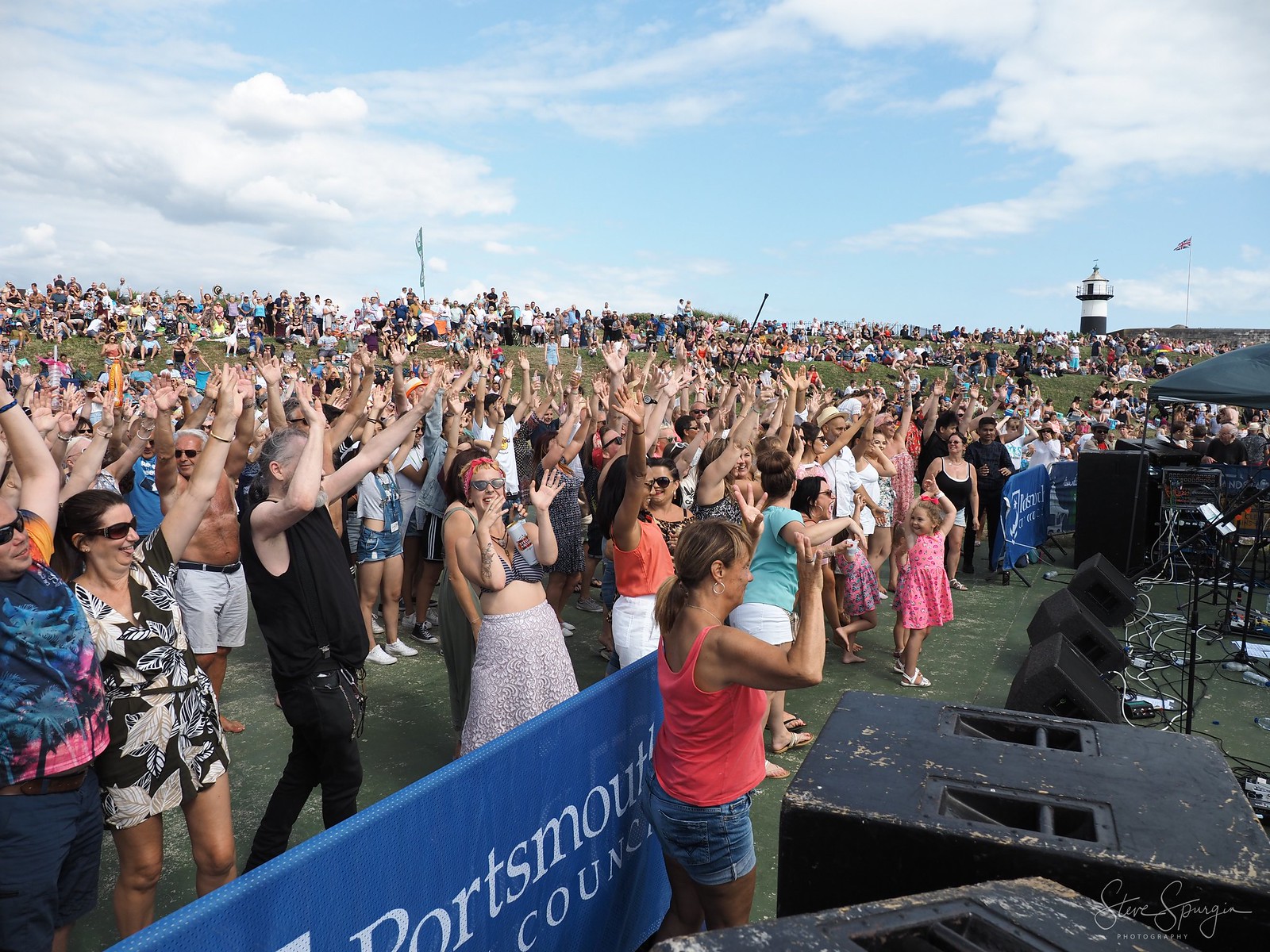The image depicts an outdoor daytime concert with a lively crowd predominantly dressed in casual attire. The scene is filled with smiling, laughing, and waving concertgoers, many with their hands raised in the air, creating a sense of unity and enjoyment. The audience stretches out across a flat area and up a green hillside in the background, suggesting a large gathering. On the right side of the image, there's a significant amount of musical and electrical equipment, including multiple speakers, microphones, and amplifiers, set up under a pop-up tent. In the foreground, three speakers for vocalists are visible, along with two larger black speakers on either side. A blue barrier, likely indicating the stage area, features a banner that reads "Portsmouth Council." In the distance, a black-and-white lighthouse and a flagpole with a flag can be seen against a light blue sky adorned with various cloud formations. The image has a signature in the bottom right corner, possibly reading "Steve Something Photography."